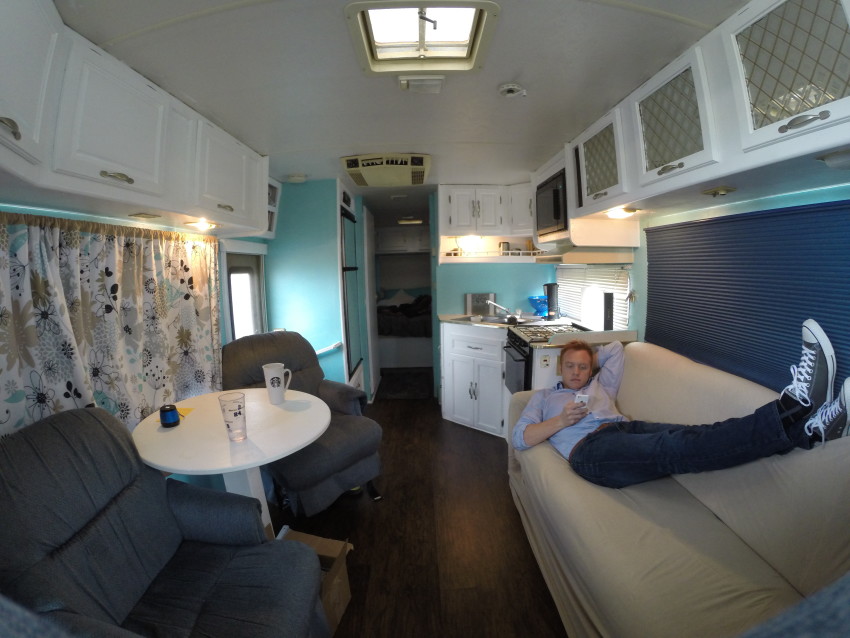In this image, we see the interior of a renovated older RV or travel trailer with a long and narrow layout. The walls are painted a pastel, powder blue, and the ceiling and cabinetry are white, giving the space a bright and airy feel. There is a noticeable yellowing of the plastic frame around the roof hatch and the cover of the roof AC unit, indicative of the RV's age. 

The scene shows a man comfortably lounging on a beige (or tan) sofa located on the right side of the frame. He is dressed casually in a blue dress shirt, jeans, and Converse sneakers, with his feet propped up as he focuses on his phone. 

To the left of the sofa, there are two dark blue armchairs positioned around a small white table that has a mug and a glass on it. Behind the man is a compact kitchen area featuring white cabinets, a stainless steel sink, and black appliances, including a stove and microwave. In addition, floral-patterned blinds are visible, adding a touch of decoration to the space.

The flooring appears to be brown hardwood, and the perspective suggests a view from the front of the RV looking towards the back, where a hallway leads to a bedroom. Overall, the space seamlessly combines living and kitchen areas, maintaining a cozy and functional atmosphere.